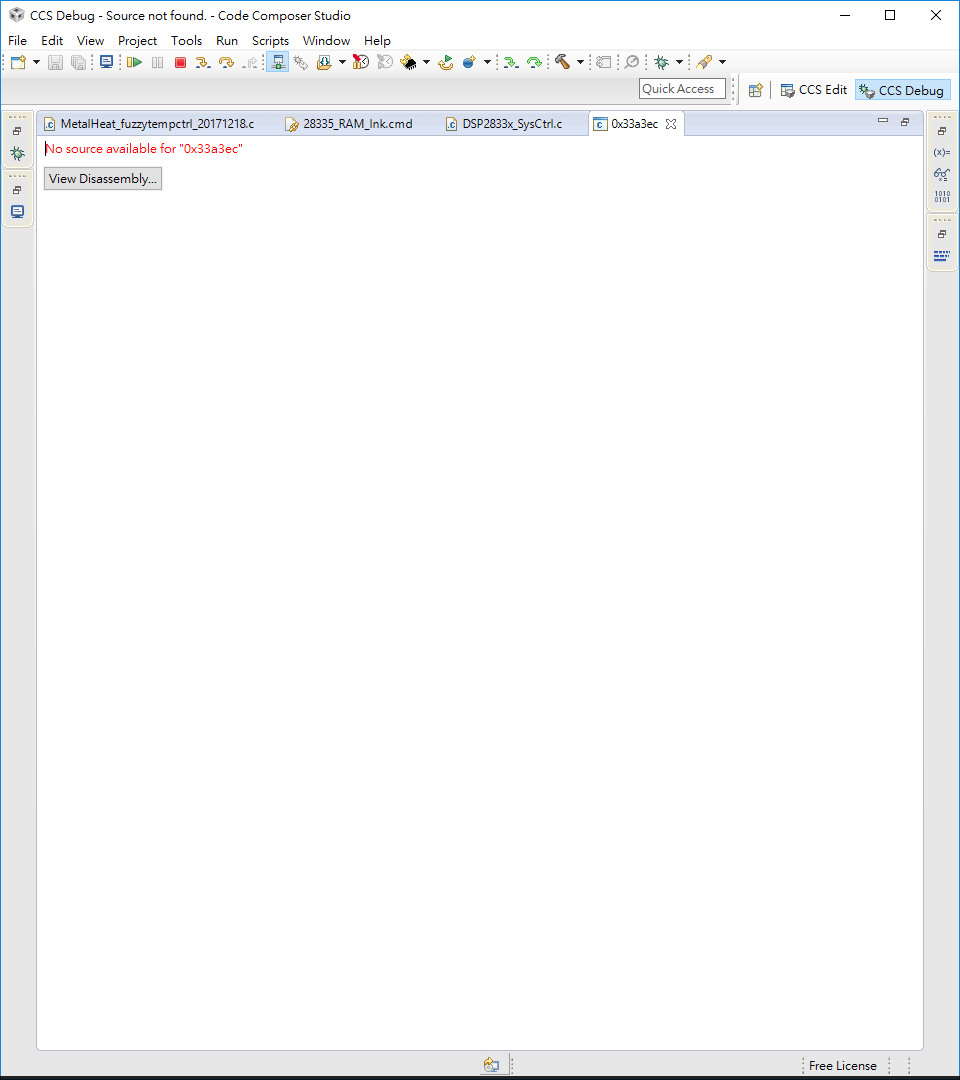The image showcases a screenshot of a software interface, specifically Texas Instruments' Code Composer Studio (CCS). At the top of the interface, the title bar prominently displays "CCSDebug-SourceNotFound-CodeComposerStudio." Directly below this, a series of drop-down menu options are visible, including "File," "Edit," "View," "Project," "Tools," "Run," "Scripts," "Window," and "Help." 

Below the menu options, there's a toolbar filled with various icons. Some of these icons depict a file folder, a green arrow pointing to the right, a yellow downward arrow, a hammer, and a rocket, among others, suggesting a range of functionalities like file operations, debugging, building, and running projects.

Further down, another row features a search bar labeled "Quick Access." Beside it, there are tabs named "CCS Edit" and "CCSDebug," both accompanied by icons.

On the left side of the screen, a vertical toolbar includes four icons representing different tools or views, such as a debug tool, a computer monitor, among others.

The main workspace of the interface is divided into columns displaying different text files and messages. The listed files include "MetalHeatFuzzyTempControl20171218.c," "28335_RAM_LNK.cmd," and "DSP2833X_SYSCTRL.c." Additionally, a hexadecimal address "0x33A3EC" is shown, accompanied by an adjacent 'X' symbol. 

A prominent red message indicates, "No Source Available for 0x33A3EC," alerting the user to a missing source file. Below this message, there is a clickable box labeled "View Disassembly," offering an alternative way to inspect the code at the given address.

This detailed layout highlights the functionalities and current focus areas within the Code Composer Studio development environment.